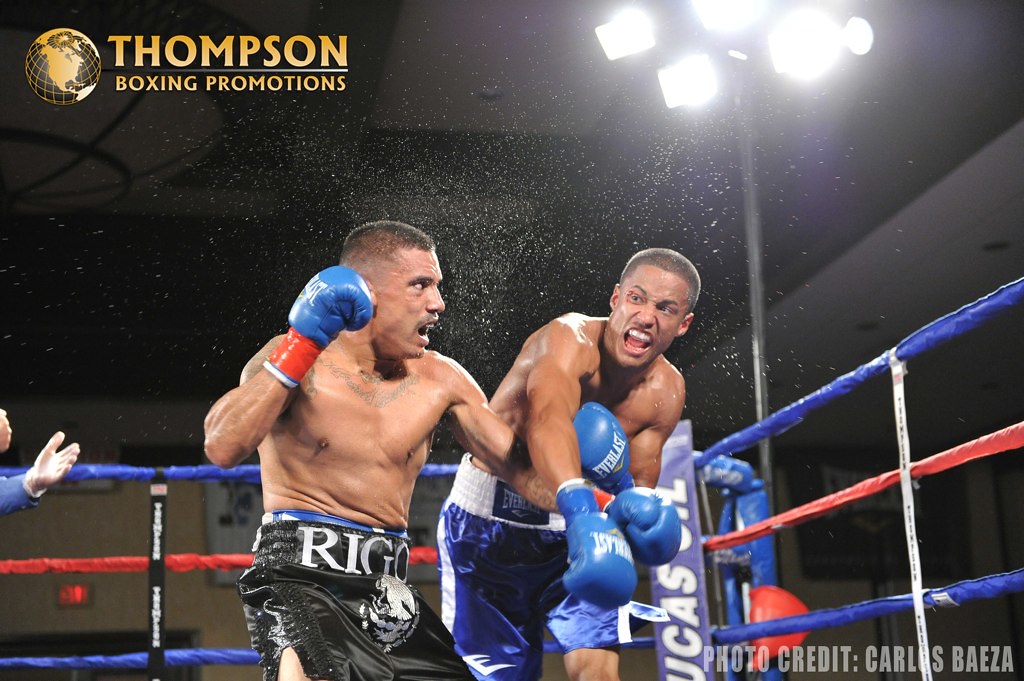In this photograph capturing a vibrant indoor boxing match, two African-American men are the focal points, engaged in an intense bout. Inside the boxing ring, enclosed by red and blue ropes, the man on the left is wearing black trunks adorned with the name "RIGO". His blue-gloved fist is raised, and his mustached face is caught mid-shout. Opposite him, the man on the right, clad in blue trunks, is lunging forward post-punch, his mouth also open, and sweat flying off both fighters, capturing the high-octane moment. To the left, a blue-shirted referee’s hands are partially visible. The top left corner of the image bears the golden words "Thompson Boxing Promotions" alongside a globe graphic. Above the boxers, a mounted pole with four illuminating lights brightens the scene, emphasizing the electrifying atmosphere of the match. In the bottom right corner, the photo credit reads "Carlos Baeza".